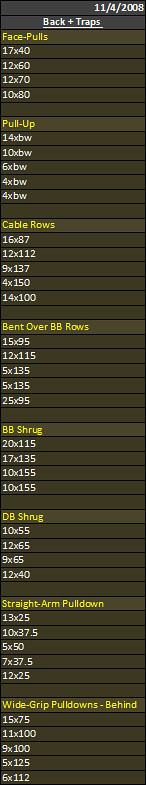This image shows a detailed, vertically oriented workout chart dated 11-4-2008 at the top left corner. The chart's heading reads "BACK + TRAPS" and outlines a structured exercise regimen. The background is brown, and the chart is divided into various sections, each dedicated to a specific exercise. 

From top down, the exercises listed include:

- **Face Pulls**: Noted in yellow with repetitions such as 17x40, 12x60, 12x70, 10x80.
- **Pull-Ups**: Also noted in yellow with varying repetitions like 14xBW, 10xBW, 6xBW, 4xBW.
- **Cable Rows**: Entries include 16x87, 12x112, 9x137, 4x150, 14x100.
- **Bent Over Barbell Rows (BB rows)**: Repetitions listed are 15x95, 12x115, 5x135, 5x135, 25x95.
- **BB Shrug**: Noted with entries like 20x115, 17x135, 10x155.
- **DB Shrug**: Listed repetitions are 10x55, 12x65, 8x65, 9x65, 12x40.
- **Straight Arm Pull-Down**: Listed as 13x25, 10x37.5, 5x50, 7x37.5, 12x25.
- **Wide Grip Pulldown Behind**: Repetitions include 15x25, 11x100, 9x100, 5x125, 6x112.

Each exercise section specifies the number of sets and weights or repetitions to be performed, providing a comprehensive guide for the workout session focused on back muscles and trapezius.